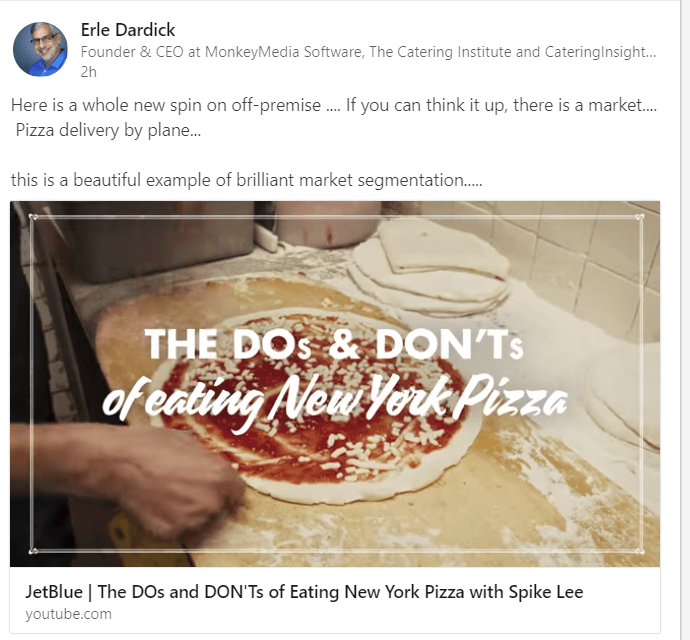At the top of the image, there is a thin gray line running horizontally across the frame. On the far right-hand side, a thicker gray line descends vertically, intersecting with another horizontal line. Upon closer inspection, a thin gray border can be seen partially framing the image on the right side before disappearing entirely.

At the top section of the image, there is a circular profile picture set against a bluish-gray background. The profile picture features a man with salt-and-pepper hair wearing black glasses. He is dressed in a blue collared shirt, with a white button visible. Underneath the profile picture, the name "Earl Dardick" is written in black text. Below his name, in slightly smaller black text, it reads "Founder, The Ansible, CEO at Monkey Media Software, The Catering Institute, and Catering Insight." To the right of this, "2H" signifies that this information was posted two hours ago.

Beneath this, there is a text block that reads, "Here's a whole new spin on on-premise. If you can think it up, there's a market. The piece of delivery by plane. This is a beautiful example of brilliant market segmentation."

The main image is a rectangular photo showing a circular pizza base with sauce and toppings. Above the pizza photo, in white text, it says, "The Do's and Don'ts of Eating New York Pizza." Below this text block, there is a line that reads, "JetBlue: The Do's and Don'ts of Eating Pizza with Spike Lee," followed by a link to a YouTube video: "youtube.com."